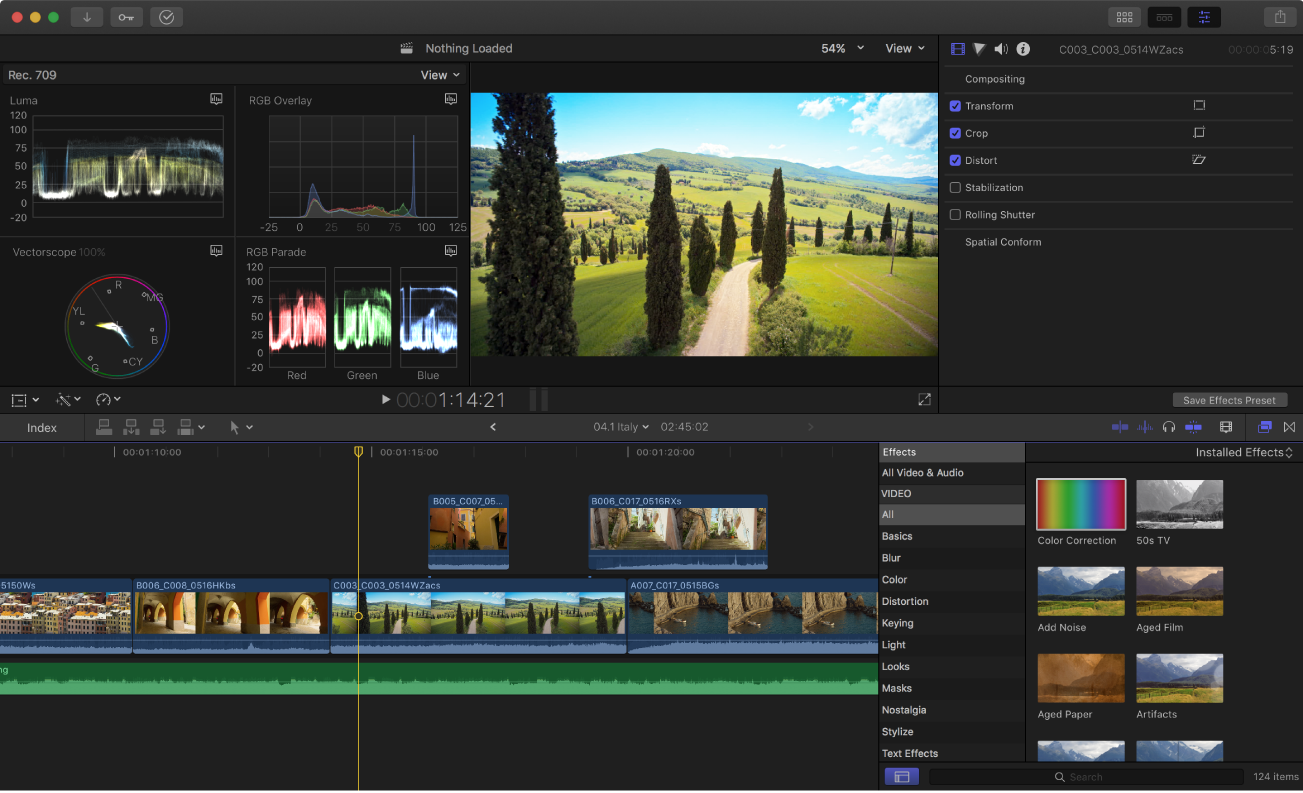The image depicts a detailed screen capture of a video editing software interface, possibly Adobe Lightroom, with various editing tools and previews visible. Central to the screen is a captivating landscape showing a blue sky overhead adorned with white clouds. The picturesque scene features verdant hills and lush green fields, flanked by towering cypress-like trees on either side of a dirt road or pathway. The bottom part of the screen showcases multiple small previews of the image with different color patterns and tones, illustrating the software's versatile editing capabilities. The layout resembles that of an OBS engine screen, emphasizing the comprehensive editing functions available for adjusting brightness, color, and other visual elements of the video or image.